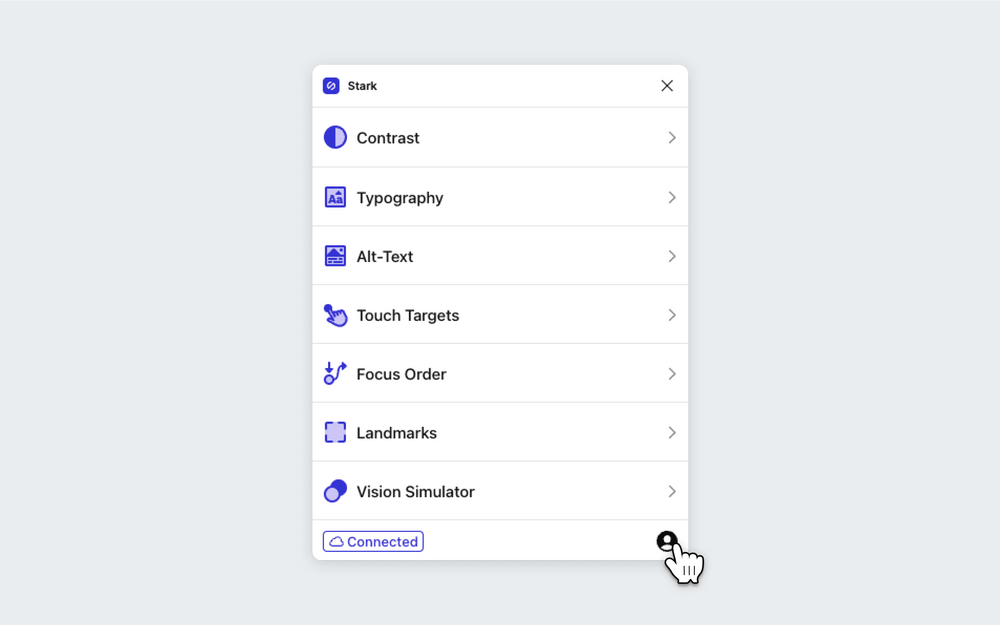This image is a detailed screenshot of the "Stark" application, likely designed for a PC despite its mobile-friendly interface. The overall layout is characterized by a clean design consisting of shades of blue and light gray. 

At the top of the screenshot, "Stark" is displayed in small lettering beside an icon that resembles the Slack logo. An "X" at the top right corner suggests that this could be a window or modal that can be closed. 

Below the title, there are several categorized sections, each represented by its own distinct bluish icon. These categories include "Contrast," "Typography," "Alt Text," "Touch Targets," "Focus Order," "Landmarks," and "Vision Simulator." Each section features an arrow pointing to the right, indicating that they can be expanded or navigated into for further options or settings.

In the bottom right corner, a person icon signifies the account login status, typical for applications requiring user authentication. The bottom left features a small blue rectangular box with a cloud icon and the word "connected," indicating that the user is currently connected to the cloud, ensuring data synchronization and backup.

Overall, this organized layout suggests that Stark is a comprehensive tool, likely aimed at providing various functionalities revolving around accessibility features and user interface design.